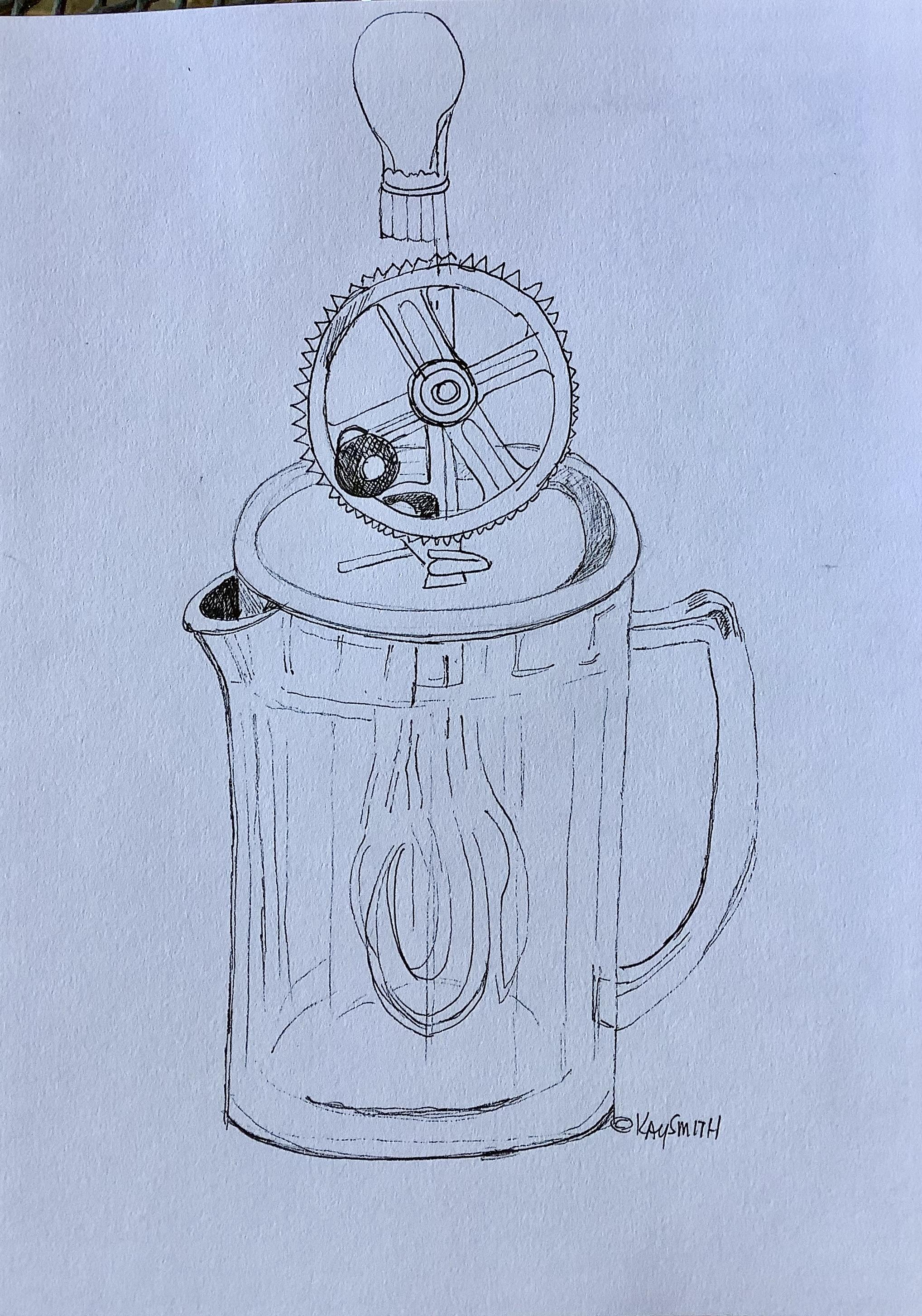This vertical rectangular image is a pencil drawing on textured paper, depicting a mechanical egg beater integrated into a pitcher. The pitcher resembles one typically used for serving beer, complete with a handle on the right and a spout on the left, giving it a potentially clear, see-through appearance. At the top of the pitcher, there's a lid featuring an egg beater mechanism with a handle shaped somewhat like a light bulb. Below the handle is a crank connected to visible gears on the side. Inside the pitcher, you can see the two beaters poised for mixing. The image is predominantly rendered in shades of black, with some light blue and faint light brown accents. The lower right corner of the drawing displays the artist’s name, "View Smith."